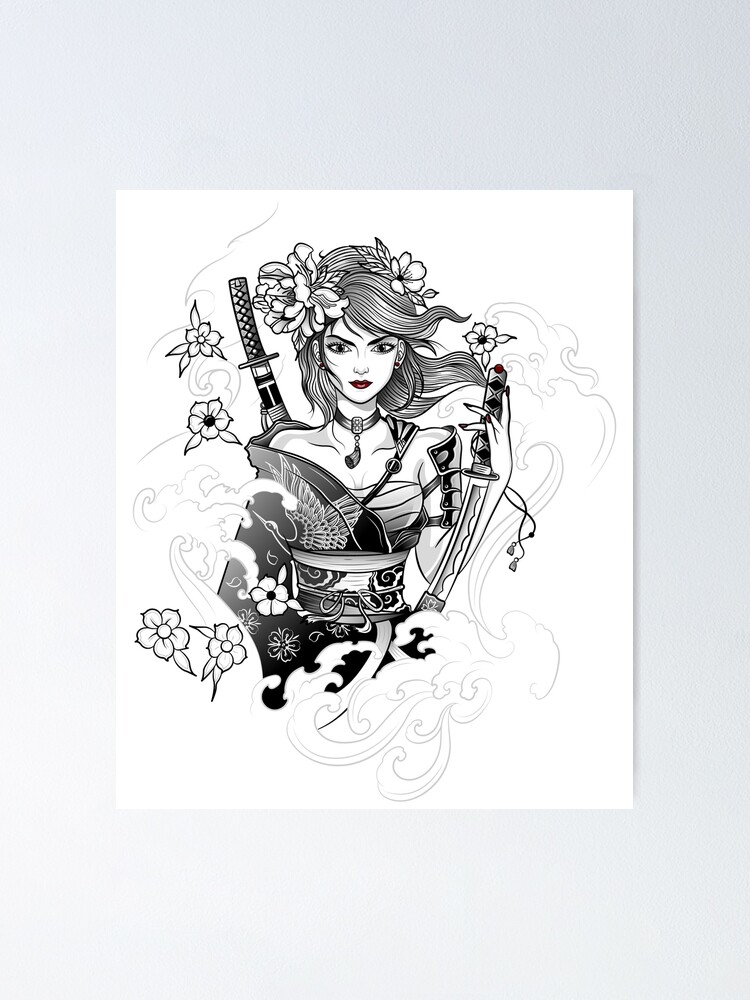The image is a vertically rectangular black and white drawing with a faint blue border that fades to white on the lower left side. At the center lies a piece of white paper against a smooth, gray background. On this paper is an intricate black ink drawing of a woman with long, flowing hair, adorned with flowers. The wind blows her hair to the right side of the image.

The woman, facing towards the viewer, wears an outfit reminiscent of a kimono that cinches at the waist and leaves her shoulders bare. She has bandages wrapped around her chest and a choke collar around her neck. Her left shoulder is adorned with armor while she pulls a knife from a sheath on her left side. A katana-style sword is strapped across her back. Her kimono features a bird design with visible feathers, adding to the detail.

Flowers surround her, emphasizing the blend of strength and fragility as she's depicted. There's an ethereal swirl of smoke around her, enhancing the conceptual feel of the artwork. Despite the image being mostly black and white, her lips are notably red, adding a striking accent to the composition. The drawing primarily focuses on her upper half, capturing the essence of a warrior in a contemplative, almost surreal scene.